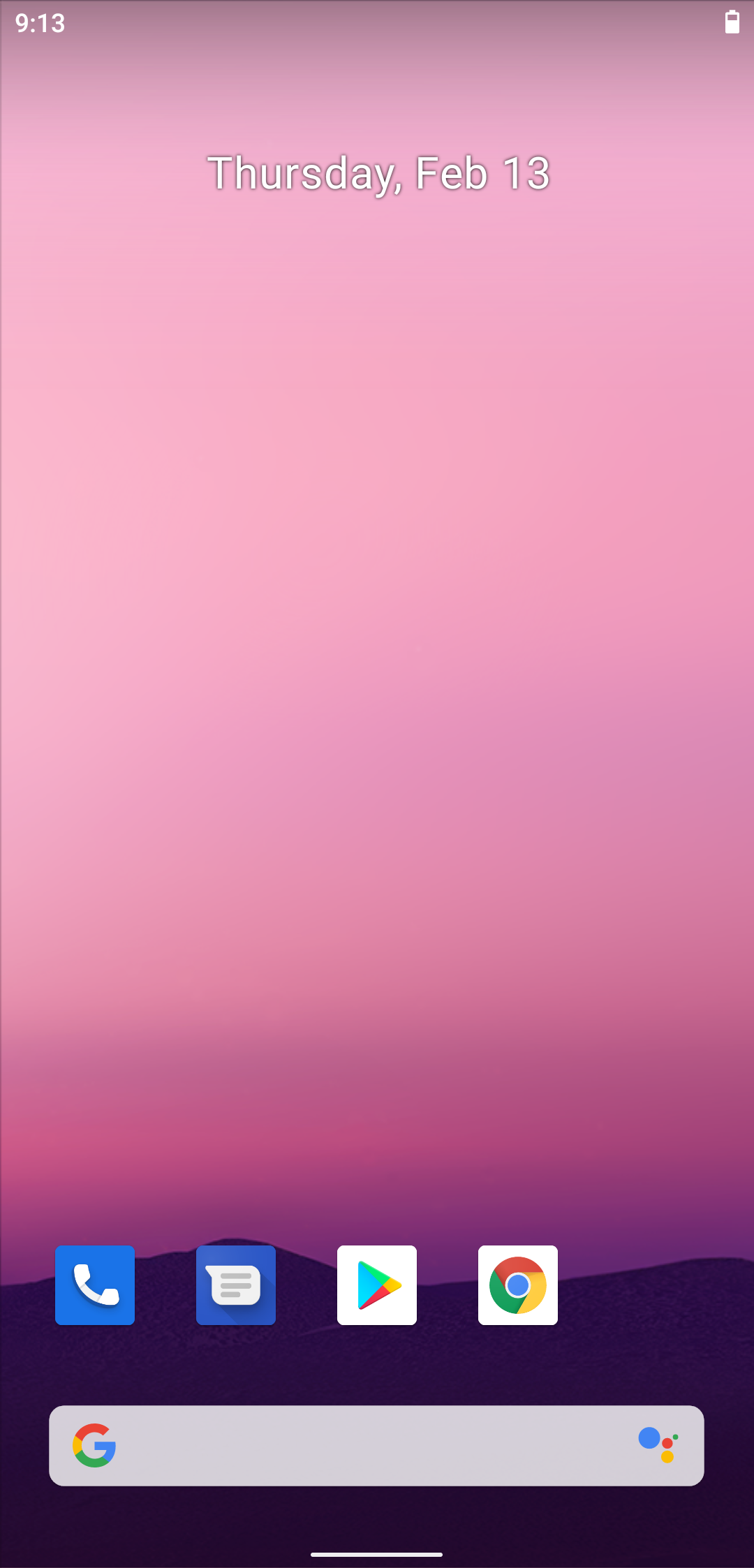The image is a screen capture of a mobile device displaying its home screen in a vertical rectangular format. The background features a gradient that transitions from a light pink at the top to a darker pink, then to a purple shade, ultimately ending in a black outline that resembles hilly terrain at the bottom. At the top of the screen, the date "Thursday, February 13" is prominently displayed in white text, and the time "9:13" appears in the upper left corner.

In the lower section of the screen, four icons are neatly arranged: the phone icon, a pop-up message bubble, the Play Store icon, and the Chrome browser icon. Just below these icons, the Google search bar is located, providing easy access for quick searches directly from the home screen. The layout and design elements suggest a visually appealing and user-friendly interface.